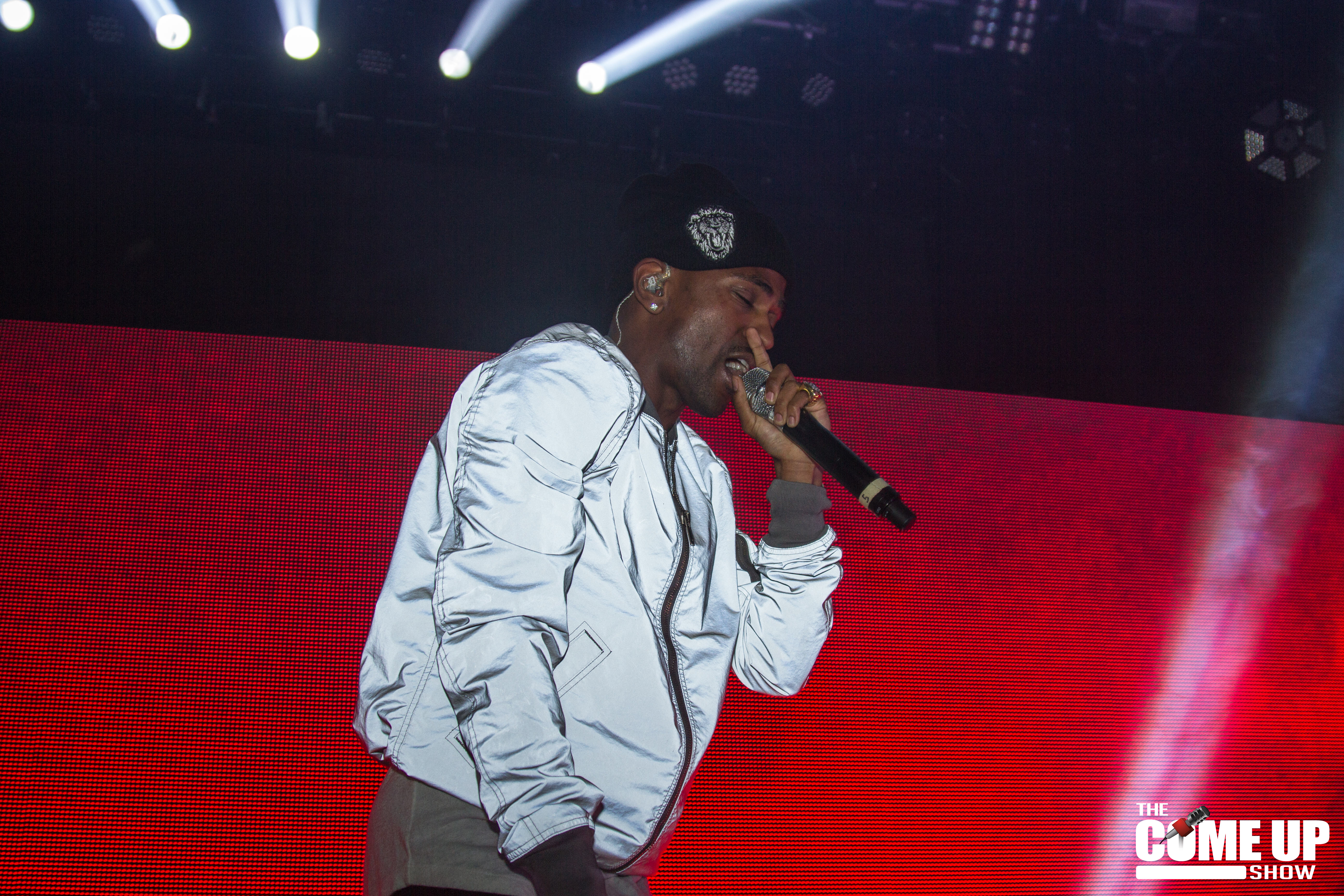This photograph captures a black man performing on stage, holding a microphone in his left hand up to his mouth. He is slightly leaning forward as he speaks or sings. The stage setup includes prominent stage lights and spotlights above him, casting beams into the audience. The image perspective is from a low angle, looking slightly upward at the man. He is wearing a black knit beanie adorned with a silver emblem, possibly in the shape of a lion. The man is dressed in a silver or reflective white zip-up jacket with brown cuffs and a beige t-shirt underneath. His gray pants are partially visible, cut off at hip level in the frame. The backdrop behind him is illuminated in red, with a black background higher up where the stage lights are mounted. In the lower right corner of the image, white text accompanied by a small microphone emoji spells out "The Come Up Show." The overall scene reflects a dynamic stage performance setting.